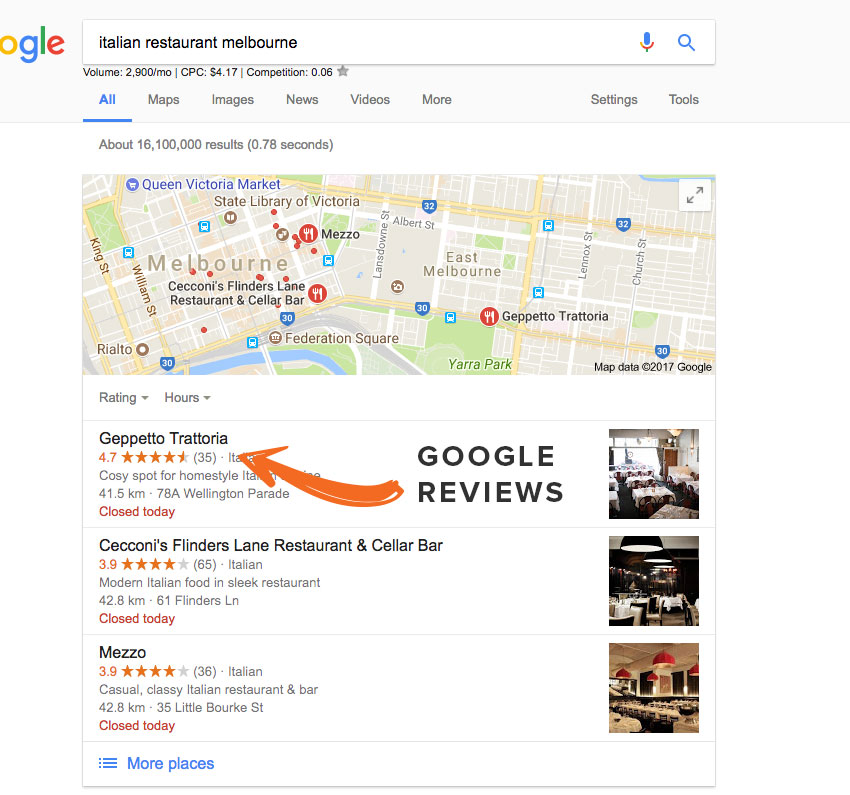This screenshot captures a Google search results page for "Italian restaurant Melbourne." 

At the top is a light gray rectangle. About two lines down on the left, you can see the Google logo, represented by an orange-gold "O," a blue "G," a green "L," and a red "E." To the right of the logo, there is a white search bar outlined in gray. Inside the search bar, in black text on the left, it reads "Italian restaurant Melbourne." To the right inside the search bar are a microphone icon and a magnifying glass icon.

Below the search bar is a blue, underlined menu bar with the following options: "All," "Maps," "Images," "News," "Videos," and "More." Further to the right, also in black text, options for "Settings" and "Tools" are visible.

Below the menu bar is a broad rectangular section. At the top of this section, there's a view that resembles a Google Map. Beneath this, on the left side in gray text, there are dropdown options labeled "Ratings" and "Hours." 

The search results list three restaurants. The first one is "Geppetto Trattoria." Below its name, in gray text, you can see a star rating, a description, and the restaurant's address. To the far right of this entry, there's a photo showing the interior of the restaurant, featuring tables with white tablecloths.

Aligned to the left of the photo, in bold black text, it says "Google." Underneath that are the word "Reviews" and a prominent green arrow pointing to a line that says "4.7" next to star icons.

Two more restaurants are listed underneath "Geppetto Trattoria," each accompanied by a picture of their respective interiors on the right side of each line.